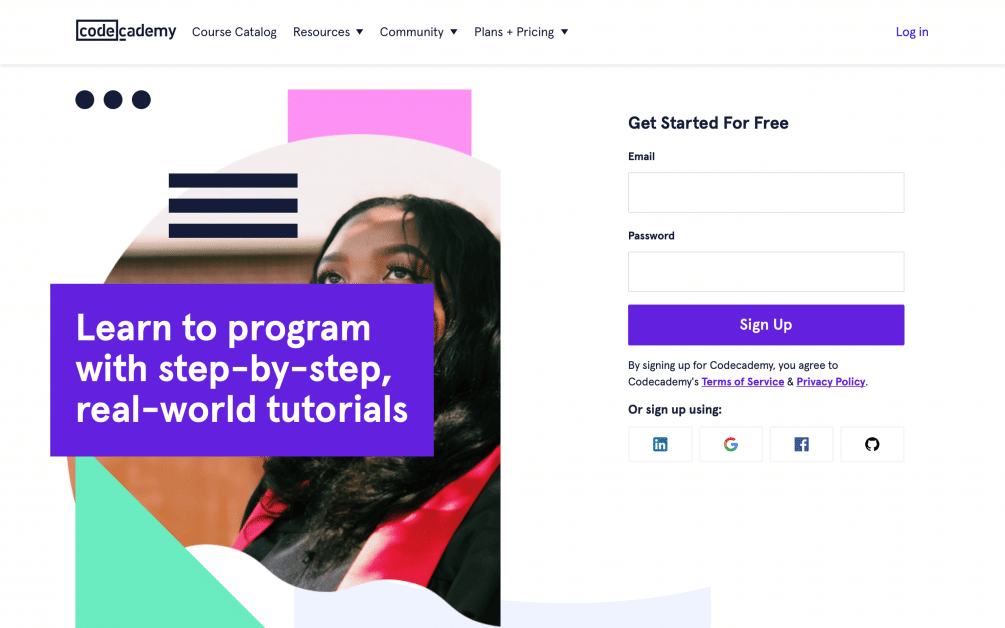The image is a screenshot from Code Academy's website. The logo prominently features the word "CODE" encapsulated within a box, followed by "cademy" in bold black letters, collectively reading "Codecademy." Surrounding the logo are navigation options: "Course Catalog," "Resources" with a drop-down menu, "Community" with a drop-down menu, and "Plans and Pricing" with a drop-down menu. Positioned in the top right corner, a small, purple "Login" link is visible.

On the left side of the image, a young Black girl is shown gazing upward, wearing a red vest. Her face is partially obscured by a large overlay text box, which prominently reads, "Learn to program with step-by-step real-world tutorials." Below this, a green triangle adds a pop of color. The background features several horizontal black bars and three dots on the left side, along with a pink bar behind the girl.

To the right of the girl's image, the text invites viewers to "Get started for free." Underneath this prompt, there are fields to enter an email address and password, accompanied by a purple "Sign-up" button. Fine print at the bottom notes that by signing up, users agree to Codecademy's Terms of Service and Privacy Policy, both of which are clickable and highlighted in purple. Additionally, options to sign up using LinkedIn, Google, or Facebook are provided, along with an unidentified fourth option depicted by a circle with white in its center.